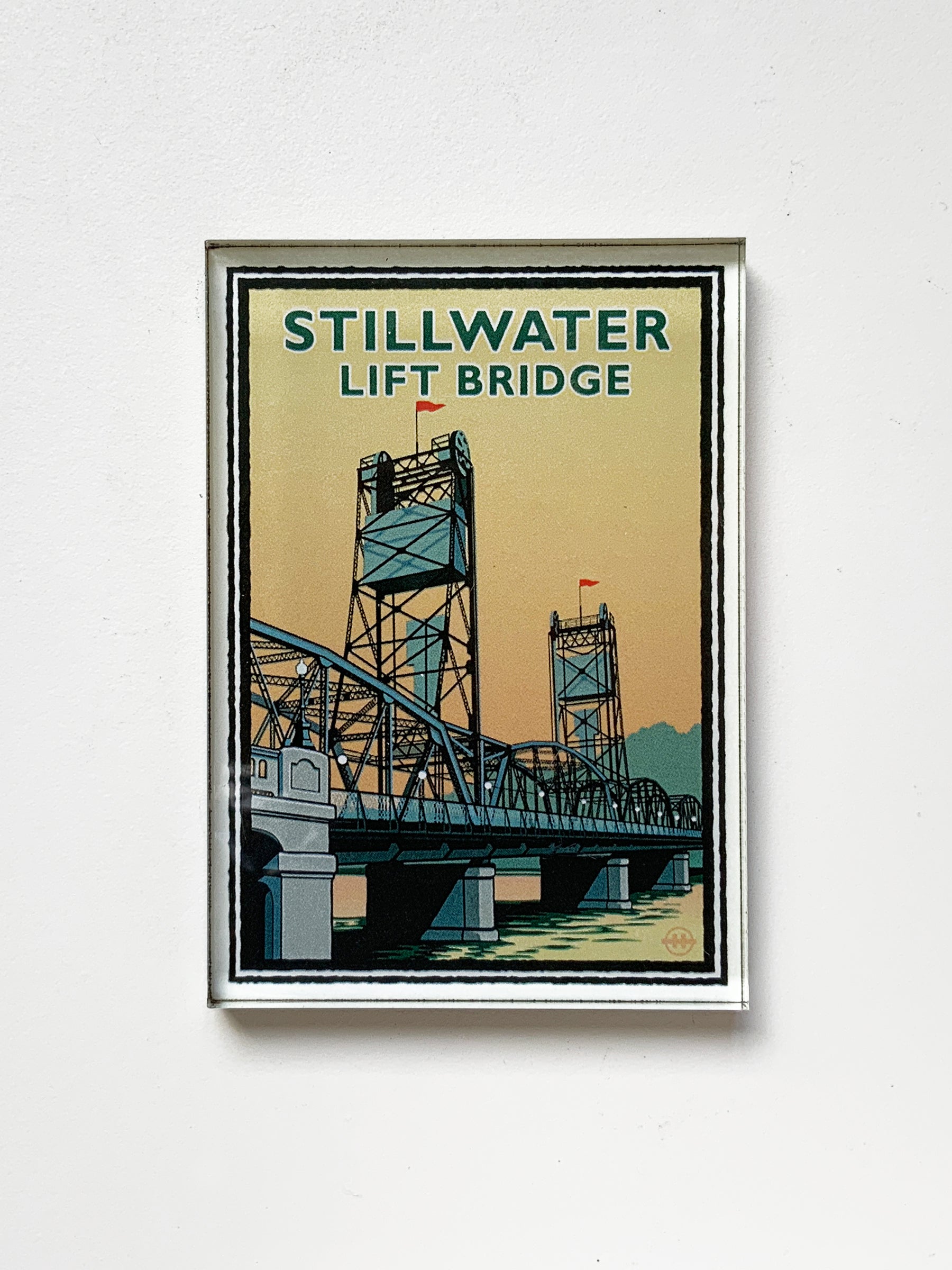The image is a vibrant, highly detailed print, framed in a white frame with a black border, and mounted on a white wall. The title, "Still Water Lift Bridge," is prominently displayed at the top-center of the print. The focal point of the artwork is a bridge painted predominantly in blue, featuring many arch-shaped structures on both sides and high metal towers at regular intervals, supporting a mechanism that lifts the center section of the bridge to allow taller boats and ships to pass beneath. Each tower is topped with a blue, box-shaped structure, a red flag or thread, and a cross-pattern linking both sides of the frame, presumably for safety signaling to aircraft. Below the bridge, there's a river with a greenish tint, reflecting the concrete supports of the bridge. In the background, lush green trees and a mountain are visible against a striking sky transitioning from yellow to orange to red and eventually to a light blue. The clear image and bright setting are enhanced by excellent lighting, making all the vivid colors and fine details easily visible.